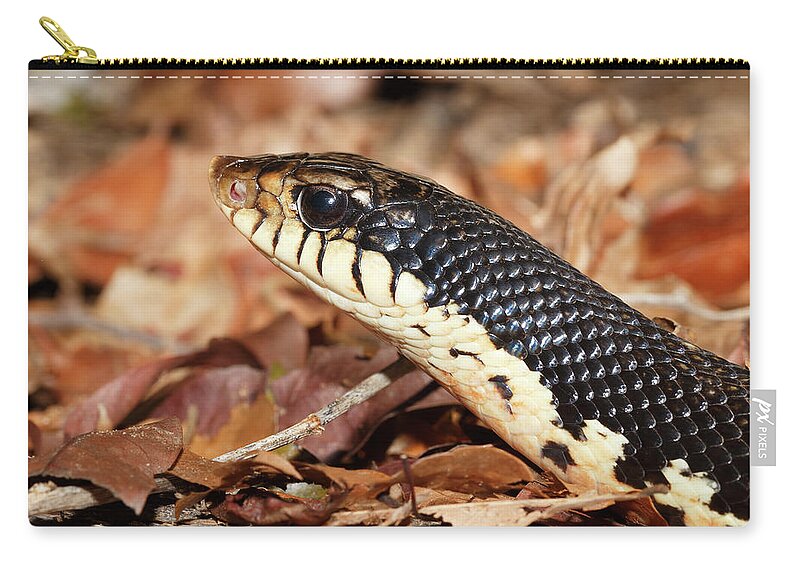This detailed image features a close-up, profile view of a snake printed on a small rectangular zip-up handbag. The snake's head, upper back, and part of its body are visible, with the snake facing left. The top of the snake is adorned with glossy black scales, while the underside is a pale ivory with black flecks. Only one dark, shiny eye is visible, highlighted with a brown accent around the iris. The bag includes a prominent gold zipper running across the top-left of the image and a distinctive stitch line underneath it. Below the zipper, a gray tag on the lower right-hand side displays the text "PX pixels" in white lettering. The background comprises a forest floor covered with dried brown leaves and scattered sticks, contributing to the photo's natural, outdoor setting.